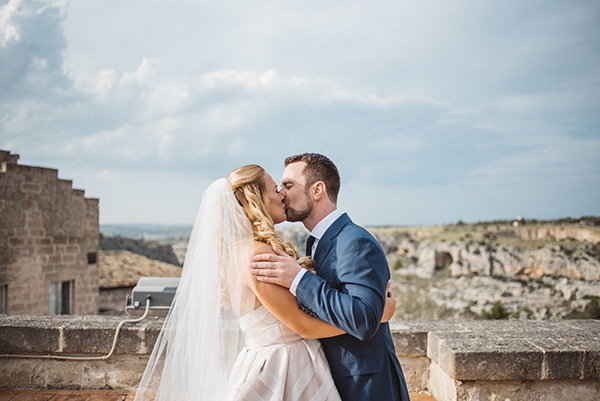In this outdoor wedding photo, a bride and groom share a kiss atop a stone or brick rooftop, creating a heartfelt moment amidst a striking backdrop. The groom, positioned on the right, is dressed in a dark blue suit and white shirt, with short brown hair and a short brown beard. He embraces the bride with one hand on her shoulder. The bride, on the left, has tanned skin and long blonde hair with the front part curly. She wears a white wedding dress and a veil pulled back from her face. Her hand is wrapped under his arm, gripping his back. Behind them, the sky is overcast but bright, illuminating their faces. The distant view features a rugged, desert-like landscape with incomplete stone structures and scattered stones, giving the scene an ancient feel. A brick building is also visible to their left, enhancing the unique setting.